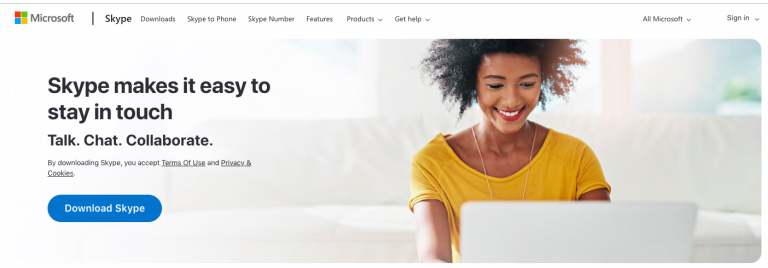In the top section of the image, a horizontal gray line spans across the width. Positioned below this line is the iconic Microsoft logo, consisting of four colored squares: red in the upper-left, green in the upper-right, blue in the lower-left, and yellow in the lower-right. The word "Microsoft" is displayed in black text next to the logo, followed by "Skype" also in black. Below these elements, the following options are listed: "Download Skype to phone," "Skype number," "Feature products," and "Get help." Towards the right side of this part, it says "Microsoft" again and includes a "Sign in" option, all within a rectangular box.

The main image to the right features a white couch partially in view, on which a woman with brown skin and curly afro hair is seated. She has bright red lipstick and is smiling warmly. She wears a mustard-colored shirt and a necklace, though part of the necklace is obscured by the top of her white laptop.

On the left side of the main image, black text reads, "Skype makes it easy to." Directly beneath this line are the words "Talk." "Chat." "Collaborate." each punctuated with a period, with the initial letters "T," "C," and "C" capitalized. 

At the bottom, bold text states, "By downloading Skype, you accept Terms of Use and Privacy & Cookies," with "Terms of Use" and "Privacy & Cookies" underlined and their initial letters capitalized.